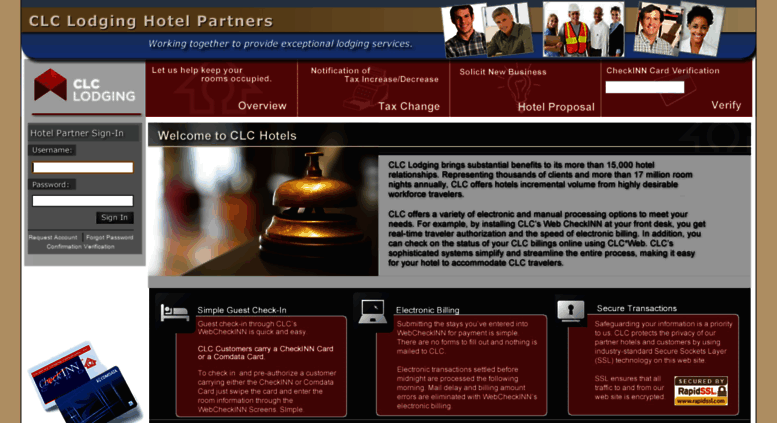**Descriptive Caption:**

The image showcases the CLC Lodging Hotel Partners website interface. In the upper left corner, there's the CLC Lodging Hotel Partners logo. Beneath it, a tagline reads, "Working together to provide exceptional lodging services." On the left side, the text "CLC Lodging" is displayed, while on the right, the text "Let us help keep your rooms occupied" is visible, followed by a detailed list that includes: "overview, notification of tax increase/decrease, tax change, solicit new business, hotel proposal, check-in (styled as INNCHECK with 'INN' in capitals), card verification." A data field for card verification is provided, labeled "verify."

On the left side of the webpage, there is a section titled "Hotel Partner Sign In," which includes data fields for username and password, accompanied by a "Sign In" button. Below this section, a welcoming message reads, "Welcome to CLC Hotels," explaining that "CLC Lodging brings substantial benefits to its more than 15,000 hotel relationships, representing thousands of clients in more than 17 million room nights annually. CLC offers hotel incremental volume from highly desirable workforce travelers." The information is set against a gray background.